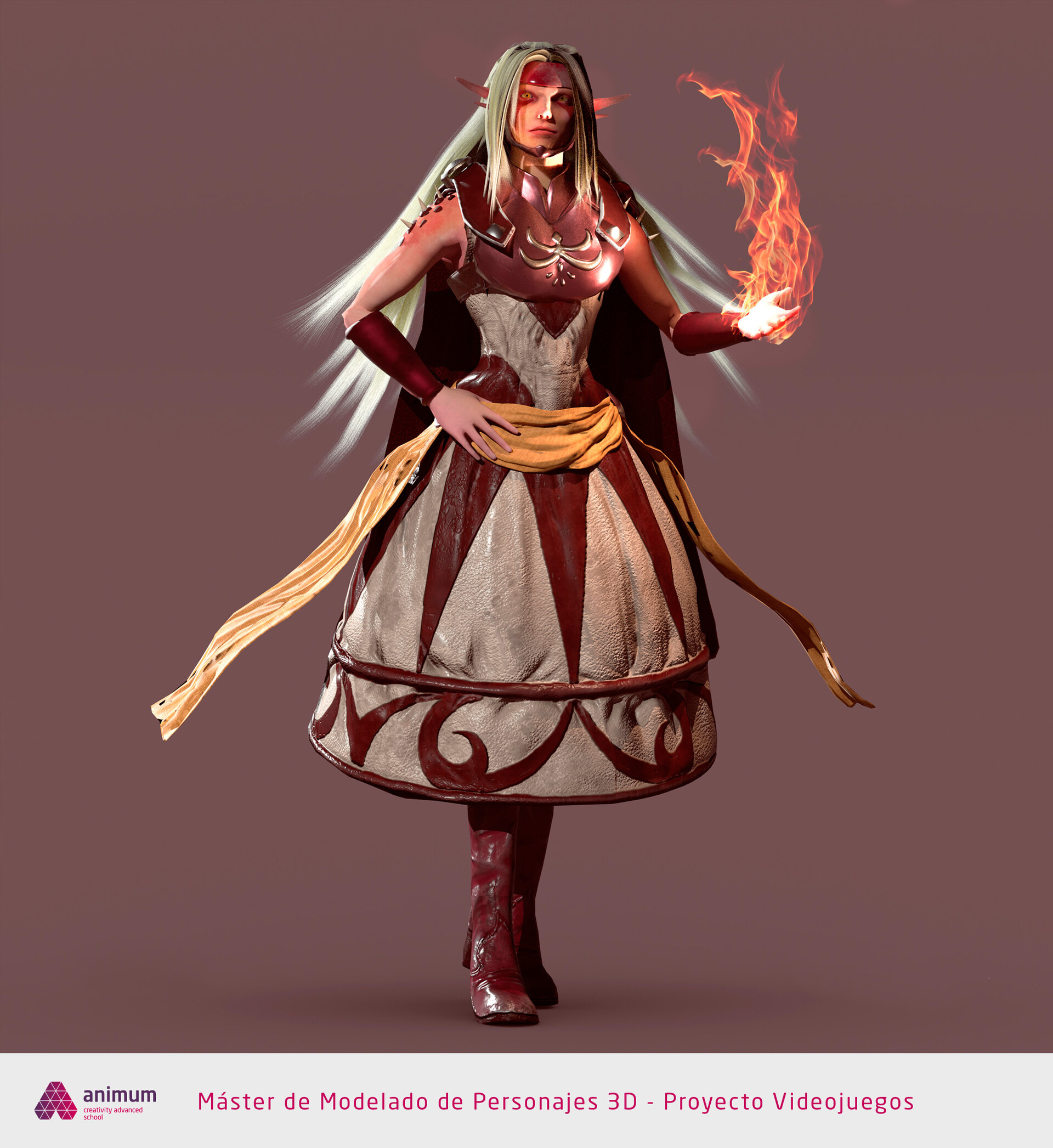The image depicts a detailed 3D anime-style digital artwork of a powerful female character, likely an elven sorceress. This striking figure boasts long, silvery-grey hair and pointy ears, characteristic of elves. She exudes a fierce warrior-like presence, donning a frock that is a blend of grey, brown, and red, accentuated with a beige sash around her waist. Her attire includes red accessories on her hands, adding a touch of vibrancy, and she is equipped with brown boots. The sorceress is depicted with blazing, orange flames emanating from her left hand, casting a warm glow and reflection on her face. The background of the image is a subtle brown or brownish-grey, providing a contrasting backdrop that highlights the character's dynamic and magical aura.